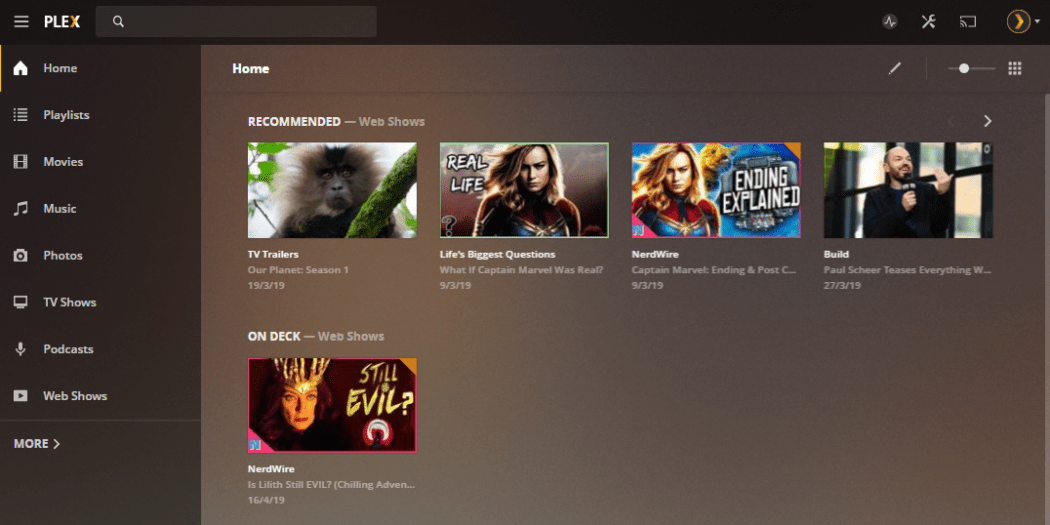Plex Interface Overview Caption:

The image portrays the Plex web interface. On the left side, a vertical menu lists various categories including Home, Playlists, Movies, Music, Photos, TV Shows, Podcasts, and Web Shows, each accompanied by a small icon. At the bottom of this menu, there is a 'More' option with an arrow pointing to the right.

At the top of the screen, a dark brown search bar with a white search icon is prominently visible. To its right, there are four small icons: a squiggly line, an 'X', two tools crossing each other in gray, and an outlined circle with an arrow pointing to the right in brown.

The central section is divided into different background colors. The darker brown area highlights the menu items on the left. The medium brown area showcases the 'Home' section prominently displayed. Below that, 'Recommended - Web Shows' lists four items:

1. **TV Trailers**: "Our Planet, Season 1" (19-3-19) featuring an ape on a branch.
2. **Life's Biggest Questions**: "What if Captain Marvel was Real" (9-3-19) featuring a female character.
3. **NerdWire**: "Captain Marvel: Ending and Post-Credit Scenes" (9-3-19) with the same female character.
4. **Build Paul**: "Sheer Teases Everything" (27-3-19) showing a partially bald Caucasian man with a microphone.

At the bottom left, under the 'On Deck - Web Shows' section, a listing for "NerdWire: Is Lilith Still Evil?" (16-4-19) is positioned, featuring an image of an ominous figure wearing a crown and captioned 'Still Evil'.